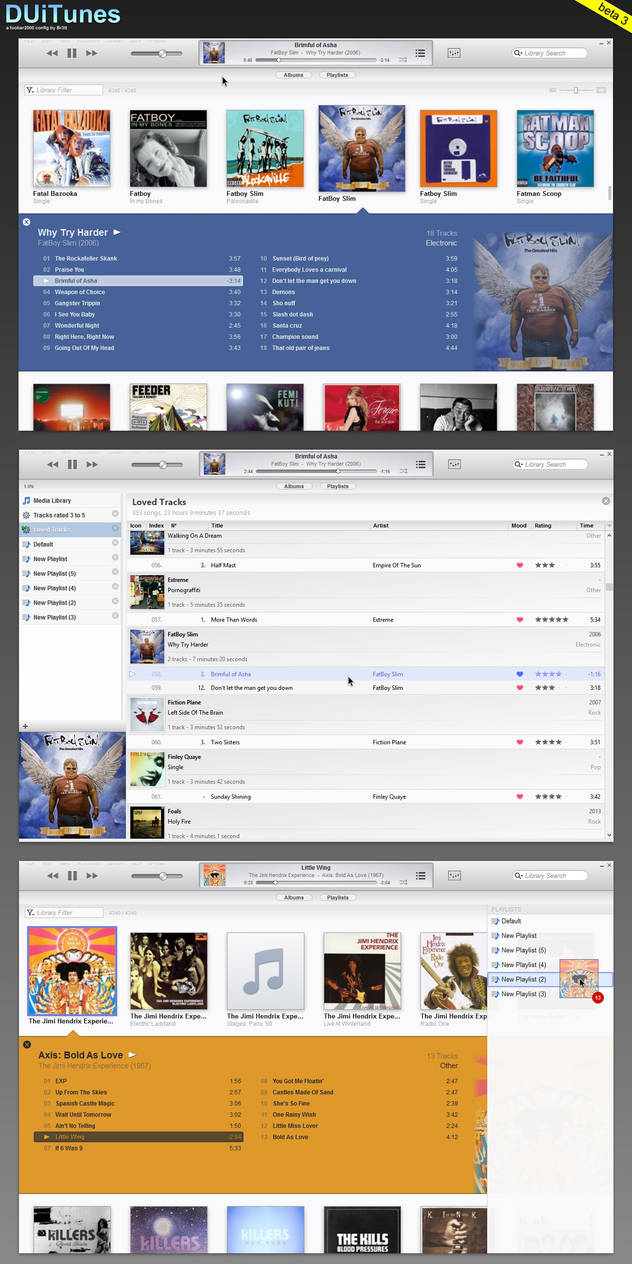The image consists of three vertically stacked screenshots of an iTunes interface, under the title "DUiTunes" with "DU" and "T" capitalized and the rest in lowercase letters. The iTunes interface depicted is a classic one with a sleek silver design. 

In the first screenshot, located at the top section of the image, the iTunes controls are visible in the upper left-hand corner, featuring buttons for rewind, fast forward, and pause, alongside a volume slider. Below these controls, there is a track list displaying the currently playing song, including its title, artist, album, and the elapsed track time. To the right of this area is a search function.

The second screenshot, found in the middle, shows a list of various album covers, prominently featuring the album "Why Try Harder" by Fatboy Slim. The selected track from this album is "Brimful of Asha," although the text is somewhat blurry and hard to decipher.

Overall, this detailed portrayal captures a nostalgic view of the classic iTunes layout, complete with album artwork and a user-friendly music control panel.